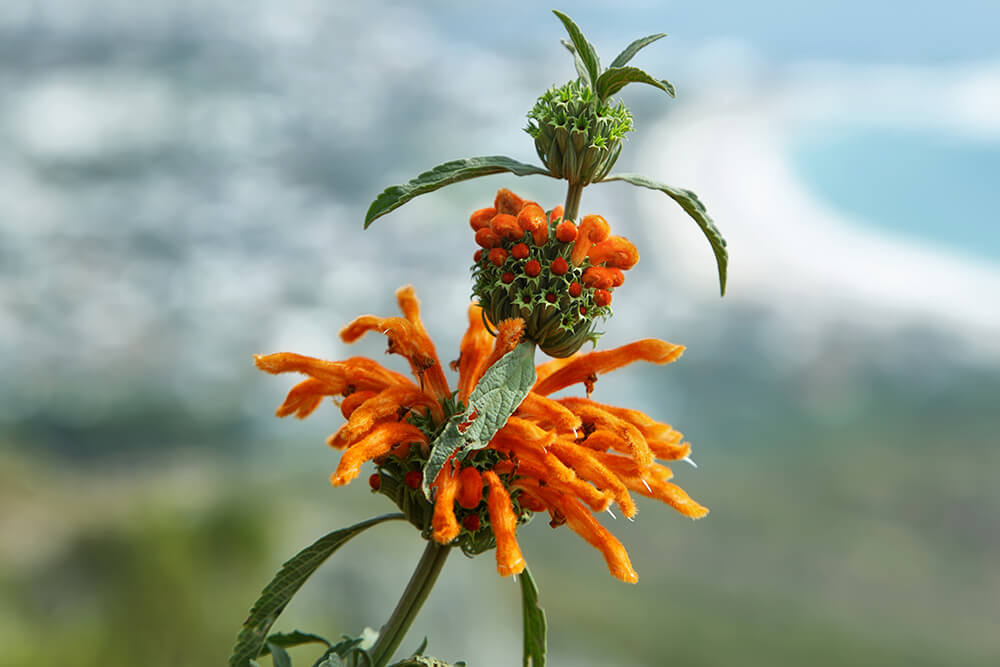The image features a striking close-up of a tropical plant with a green stem and leaves. The top part of the plant displays green leaves that have yet to bloom. The middle section is adorned with clusters of orange buds, tightly grouped like little beads. The lower part showcases prominent, vibrant tangerine-orange tube-like flowers, many tipped with white. The upper two sections seem poised to eventually produce similar tube-like flowers. The background is completely blurred, making it impossible to discern but creating a dreamy, ethereal effect that highlights the vivid, unfamiliar beauty of the plant.